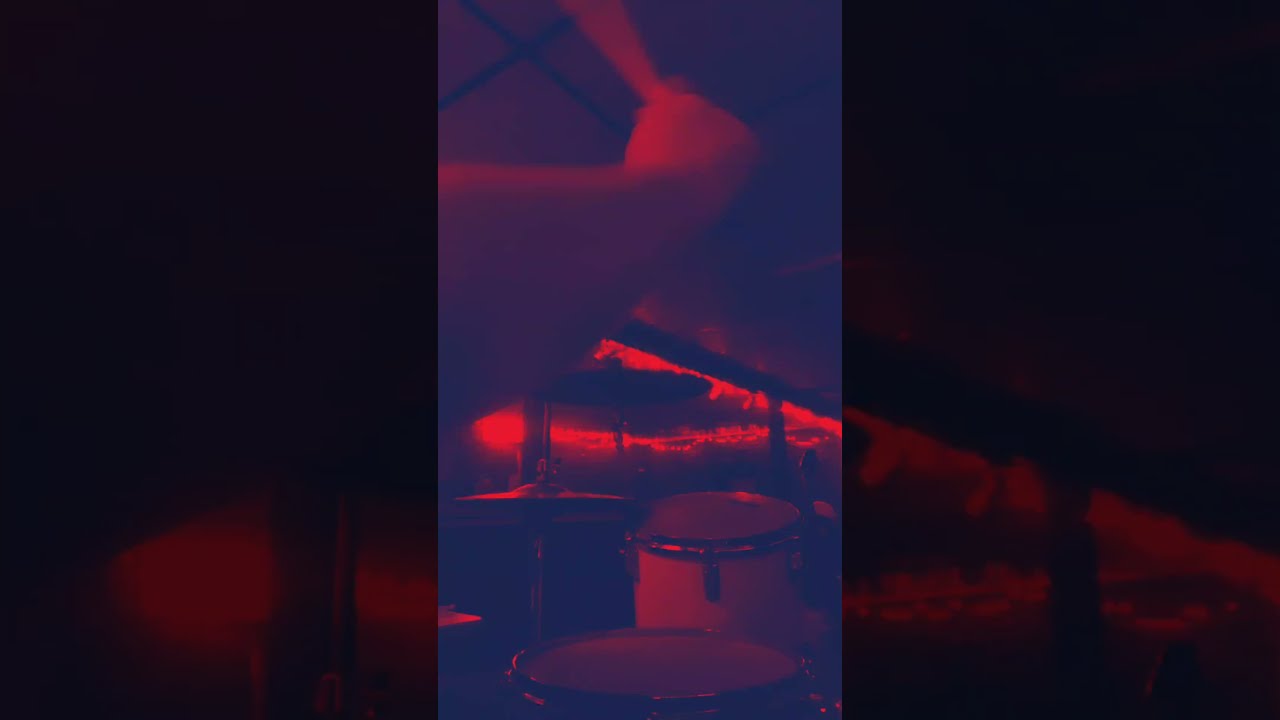In this image, we are presented with a very dark and moody scene, likely taken from a stage musical performance from the perspective of the drummer. The image predominantly features shades of dark blue and red, with a distinct reddish glow emanating from the background, resembling diffuse stage or Christmas lights. On the left-hand side, an arm is visible, holding a drumstick in a blurry motion, implying an in-action shot. The lower portion of the image reveals parts of the drum kit, including at least two drum heads and cymbals, with the entire kit being cast in a red hue. The background features a ceiling with dark lines, giving the impression of individual tiles with black gaps between them. The overall image is bathed in a bluish tint, creating an abstract, dream-like quality, as if viewed with 3D glasses that merge red and blue tones.